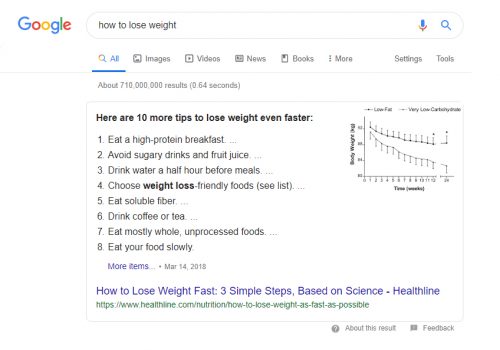An image shows a detailed Google search results page for the query "how to lose weight." Featured prominently is the search bar with a microphone search icon. The results indicate approximately 718 million entries found in 0.64 seconds. The first result presents ten tips to expedite weight loss:

1. Eat a high-protein breakfast.
2. Avoid sugary drinks and fruit juice.
3. Drink water a half hour before meals.
4. Choose weight loss-friendly tools (a list is provided).
5. Eat soluble fiber.
6. Drink coffee or tea.
7. Eat mainly whole, unprocessed foods.
8. Chew your food slowly.

Further down, the date March 14th, 2018, and a link to an article titled "How to Lose Weight Fast: Three Simple Steps Based on Science" from Healthline are highlighted. There is a small graph to the right, indicating statistical data. The image also includes a mention of www.globalonenessproject.org, although the context is unclear. The page is well-structured with sections for images, videos, news, books, and additional settings and tools.